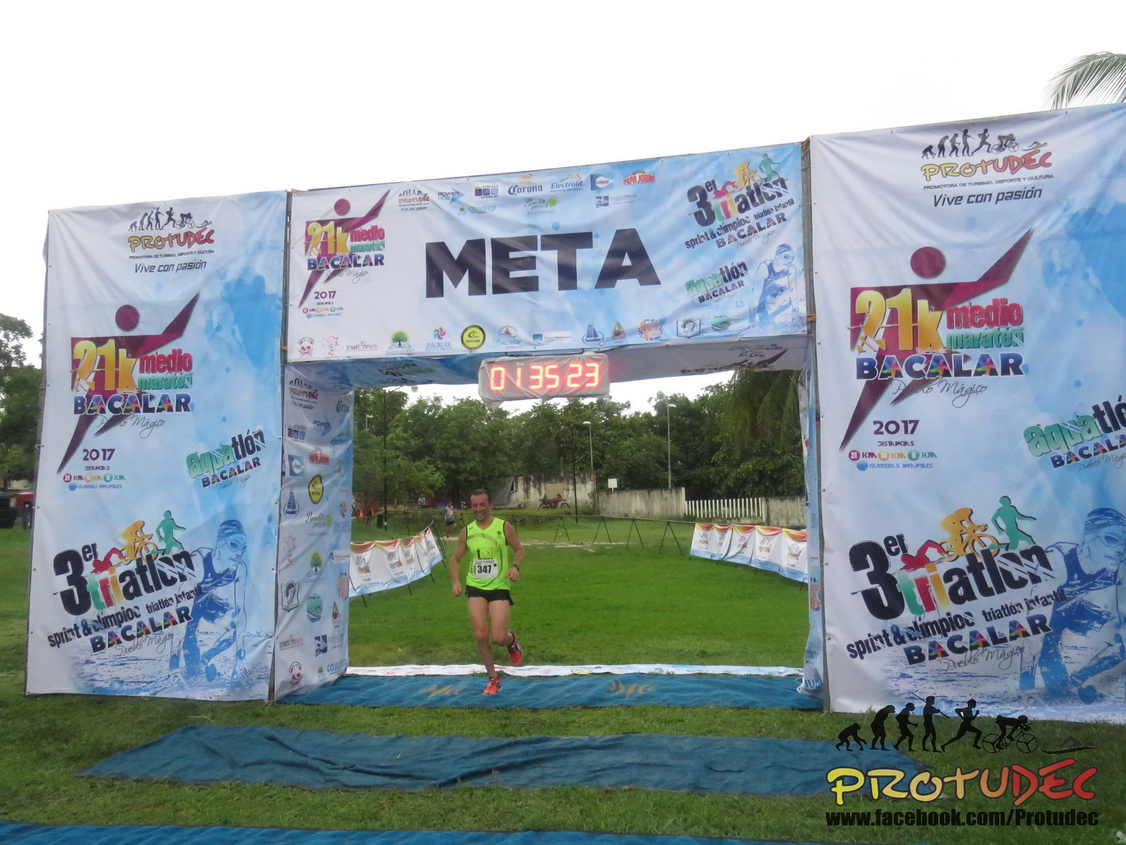In this detailed photograph, we see the finish line of a marathon race, marked by a large, square archway adorned with numerous promotional banners from various sponsors, including Metta, Protudek, Viva Compassion, Bacalar, 21K Media, and 3ER Triathlon. The word "META" is prominently displayed in dark block letters at the top of the archway. As the lone male runner, wearing a neon yellow jersey bearing the number 347, black running shorts, and red athletic shoes, crosses the finish line, the digital timer above him reads "01:35:23" in bright red and orange numerals. The scene is set on a grass-covered ground with an overcast sky and green foliage visible in the far distance. Barricades line the sides of the track, though there are no spectators present. Another runner can be seen approaching in the background. The image captures the moment with the central focus on the runner directly beneath the clock, highlighting the culmination of his race effort.